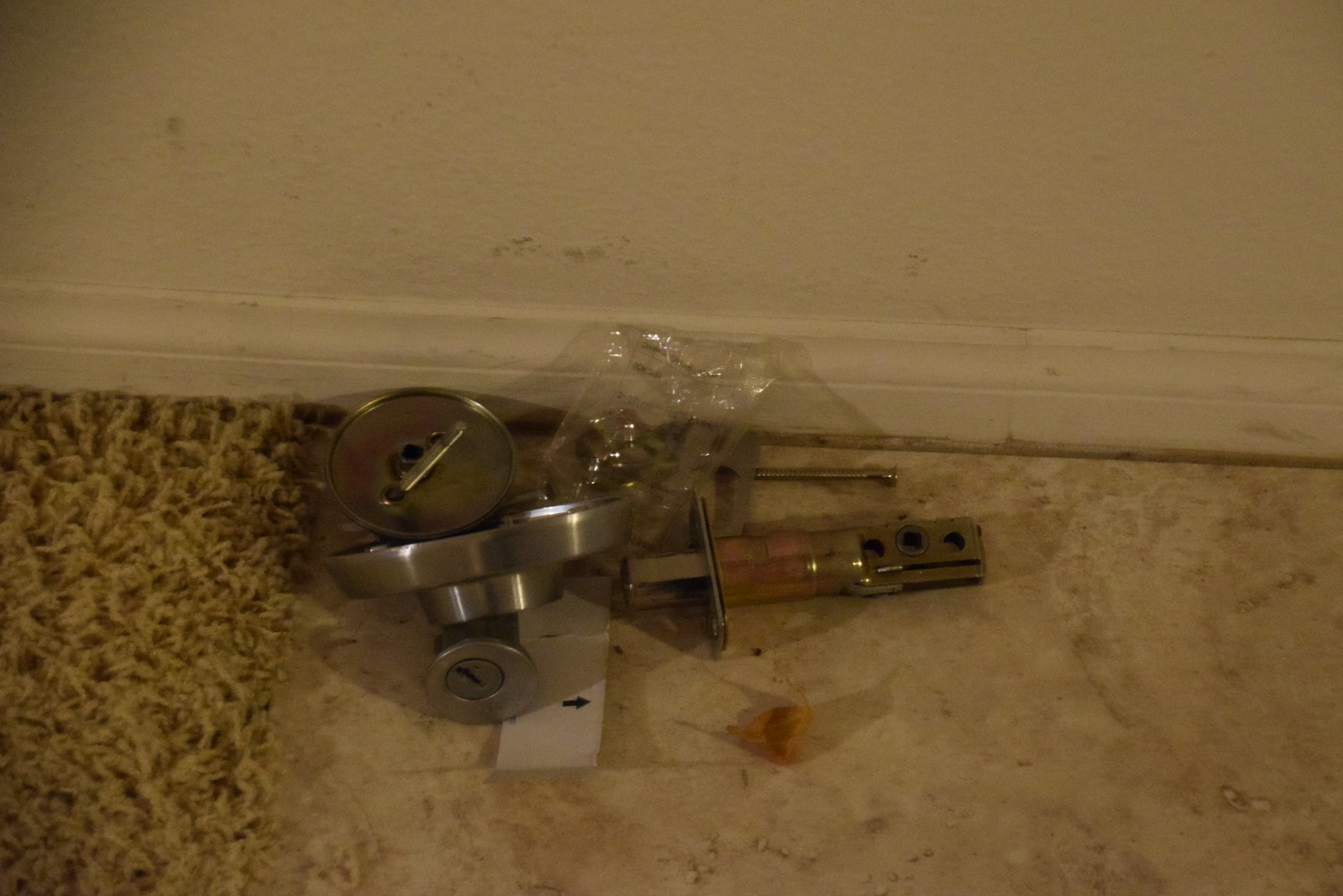The image depicts a disassembled silver metal door lock set, scattered on the floor against a white wall. The lock components, including screws, a keyhole, a metallic tube, and the deadbolt mechanism, are visibly spread out. The parts appear to have been either unpacked from a plastic bag or removed from their assembly. The flooring consists of sandy, beige-colored tiles or linoleum, transitioning into a dirty yellowish, curly carpet on the left. A shadow suggests low lighting, although the wall and wood framing remain visibly white. The scene suggests that the lock parts are being examined or prepared for installation in a household setting.